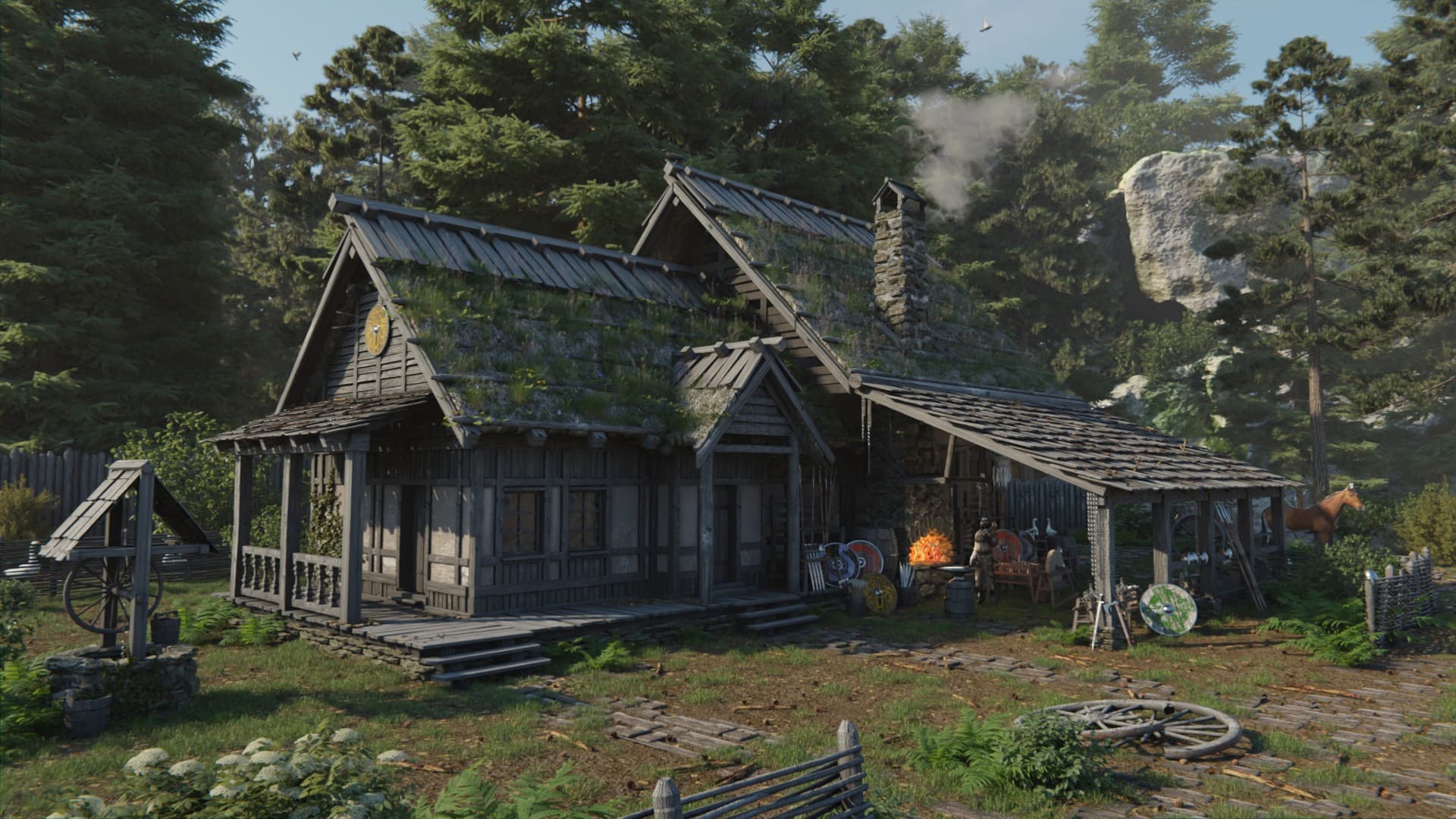The image depicts a rustic wooden house or cabin reminiscent of structures found in video games like Skyrim, Red Dead Redemption, or Elden Ring. The house showcases detailed craftsmanship, with a prominent stone chimney emitting smoke, indicating a cozy, lived-in atmosphere. The wooden roof features moss or grass growing along its side, adding to the natural, aged aesthetic. An overhang and a small front porch, accessible by three steps, add to the charm. 

Around the property, a wooden fence outlines the area, and a wagon wheel is knocked over on its side near a stone walkway leading to the house. This path also reveals several wagon wheels scattered across it. Adjacent to the house, there's a well with a bucket perched on its stone rim. There is an L-shaped side porch with two walkways leading to separate doors. Additionally, a blacksmith's forge is visible, complete with rounded shields and people tending to the forge and working on the shields.

In the background, a horse stands quietly, while trees under a blue sky and an outcropping of white rock add depth to the scene. A bright orange plant is noticeable on the right side of the house, complementing the earthy tones of the cabin and its surroundings. Overall, the scene is a harmonious blend of natural elements and detailed architectural features, bringing an immersive, game-like world to life.